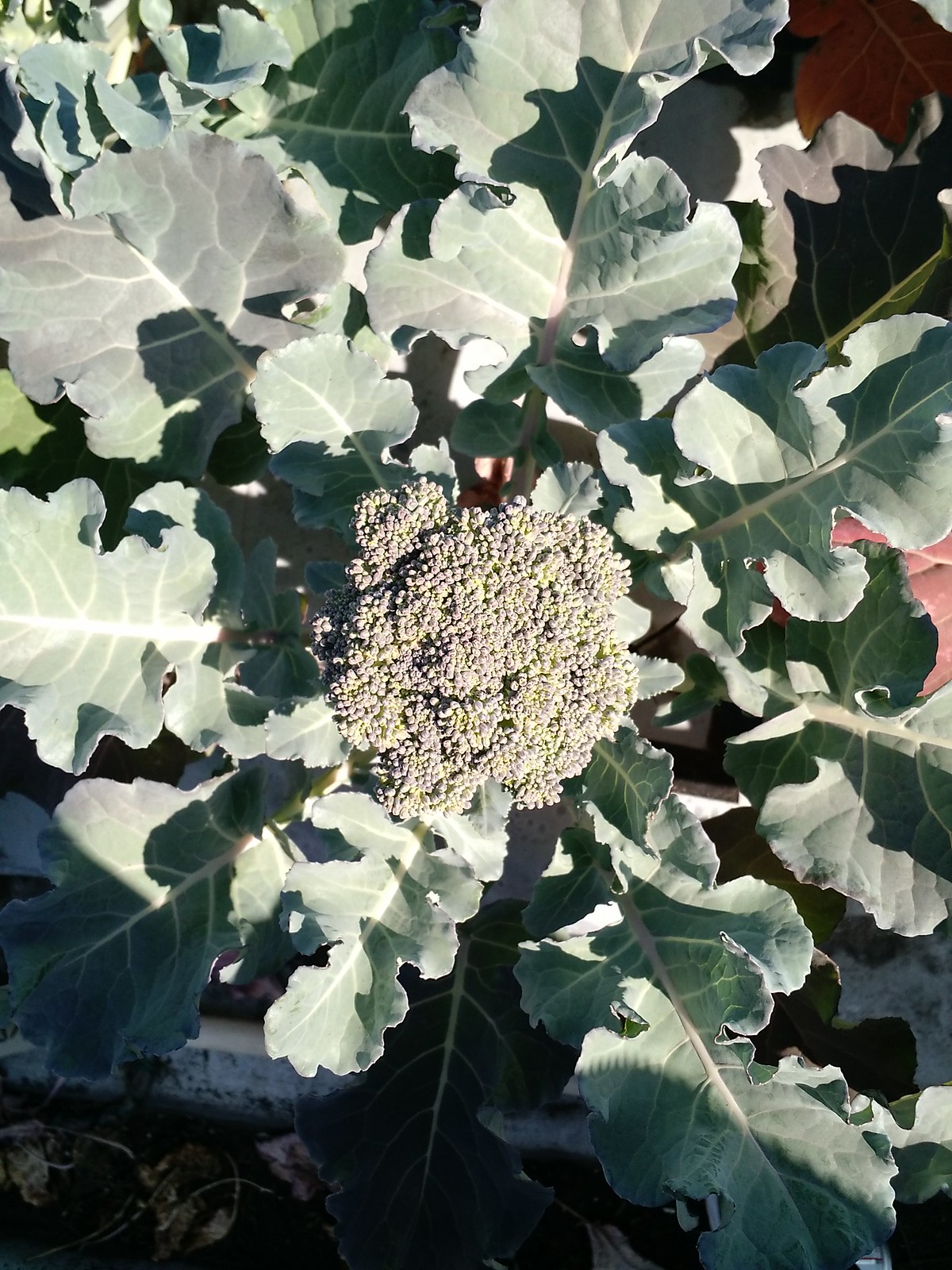The image depicts a sunny garden scene with a detailed aerial view of a broccoli plant at its center. The photograph captures large, leafy greens radiating outward. These leaves are a light green color and feature prominent, white ribbing and veins that give them a textured appearance. The sunlight is shining directly onto the plant, casting shadows on the soil and a white or silver pipe that runs horizontally at the bottom of the frame. The central floret of the broccoli is not fully matured and exhibits a mix of light green and light purple hues, along with small, clustered, seed-like formations. A hint of a red object, possibly bricks or wood chips, peeks through the leaves in the upper right corner. The overall scene combines natural elements with human cultivation, capturing the intricate details of the growing broccoli amidst its large, surrounding leaves.